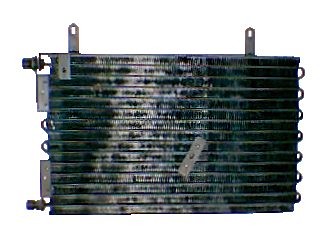This image depicts a detailed part of what appears to be a mechanical tool or possibly a piece of electrical equipment. Set against a white background, the main object is a substantial, blackish-gray structure with a ribbed appearance and multiple rivets. Horizontal and vertical lines traverse its surface, suggesting it could be akin to a filter, possibly for air conditioning or automotive use. Notable metallic elements include several silver clamps or clasps along the top of the object, each providing a reflective sheen that enhances the grayish hue in the center. The left side features additional horizontal lines and silver clasps, while the right side is lined with approximately eight hooks. The central region has a silvery, almost rectangular metal clasp or bracket, somewhat dirtied with a white fuzzy texture, possibly indicating wear. Additional features include two prominent tabs with holes at the top, potential attachment points, and some knob-like protrusions on the left. A broken tab appears to be resting in the center, hinting at a complex and well-used piece of mechanical equipment.